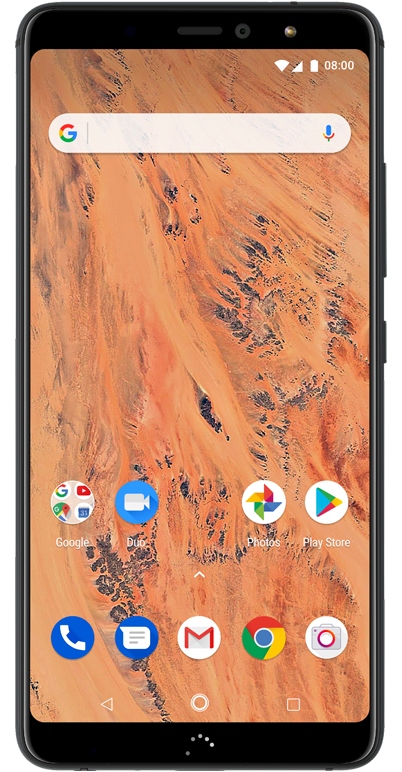The image depicts a cell phone displayed against a pristine white backdrop. The phone features a sleek black bezel, enhanced by a shiny accent stripe running along both the left and right sides. At the top center of the bezel, there's a dark grey pill-shaped speaker. Adjacent to the speaker on the right is a dark grey orb representing a camera with a black center, further accompanied by a shiny gold orb immediately to its right. 

The phone's screen exhibits a vivid home screen image that resembles an aerial photograph of a red desert, accentuated with streaks of dark grey rock formations. In the upper right corner of the screen, there are several white icons. Below them, a translucent white search bar, shaped like an elongated pill, spans the screen. On the left side of the search bar is a multicolored 'G' logo, followed by a vertical light grey separator line, and on the far right sits a multicolored microphone icon.

Further down the screen, within the negative space of the desert background, four circular icons with white text beneath them are neatly arranged near the bottom in a single row. From left to right, these icons are labeled: Google, Duo, Photos, and Play Store. Just below this row, a white arrow pointing upwards is centered. Underneath the upward arrow, there is another row featuring five circular icons. 

At the very bottom of the screen are three icons: on the left, a white outline of a triangle pointing left, in the center, two inset white circles, and on the right, a white outline of a square with rounded corners.